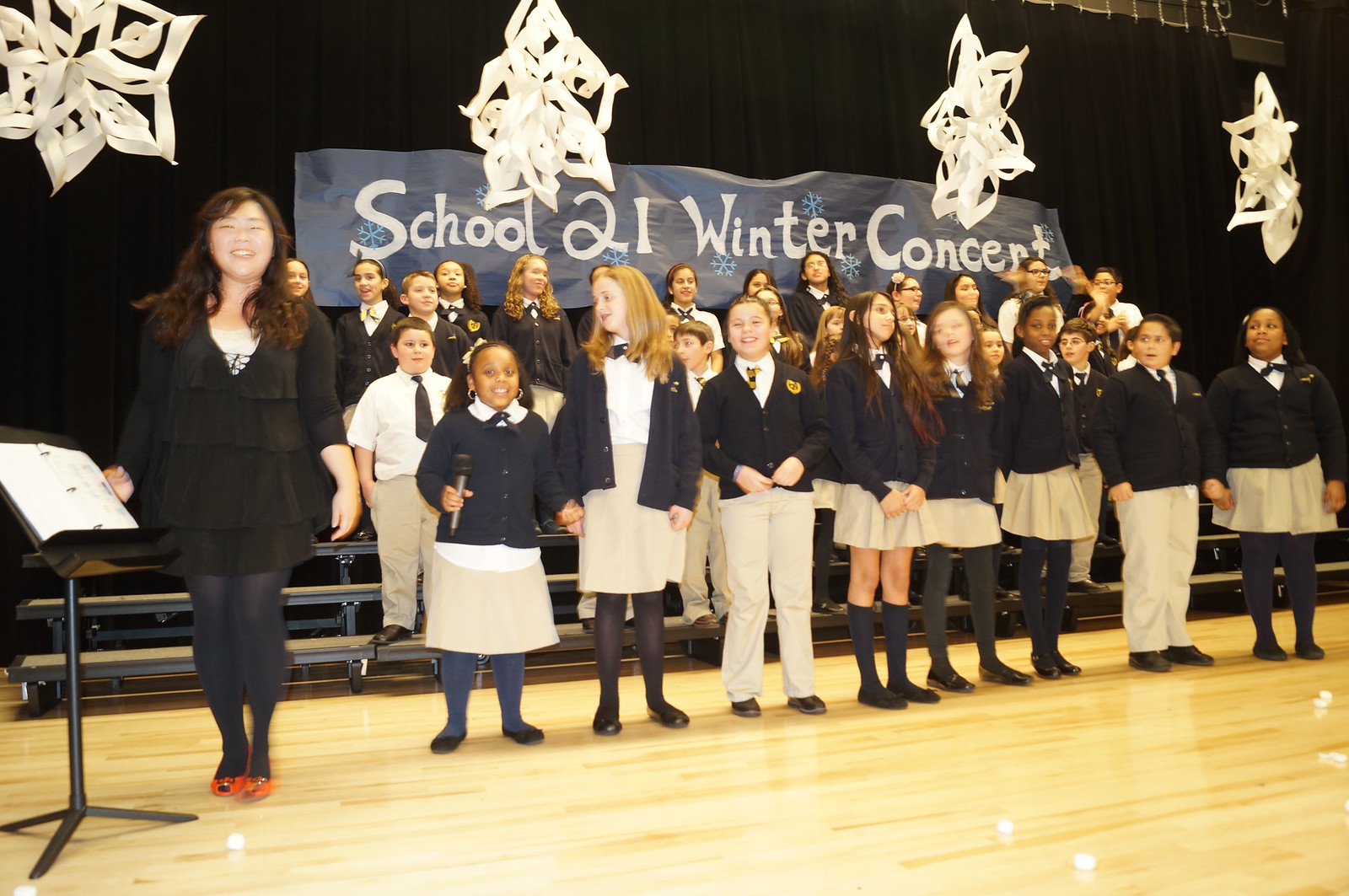The image captures a vibrant winter concert performance by children from what appears to be a private school. The children are arranged in four rows, with the back three rows elevated on bleachers and the front row standing on a wooden stage, which might be part of a basketball court. All the children are dressed in school uniforms; the boys wear black jackets with small ties, white undershirts, and khaki pants, while the girls wear khaki skirts with similar jackets. Above them, large, intricately cut paper snowflakes dangle from the ceiling, adding a festive touch. A prominent blue banner hanging above the group reads "School 2-1 Winter Concert" in white letters. Off to the left side of the children stands a teacher, likely an Asian woman, who is smiling and dressed in a black dress, red shoes, and possibly dark tights. She is positioned next to a music stand holding some material, possibly sheet music or a songbook. Her presence and the arrangement of the students suggest she plays a key role in directing the performance. The backdrop features a large black curtain, further highlighting the children's synchronized appearance and the event's formal setting.